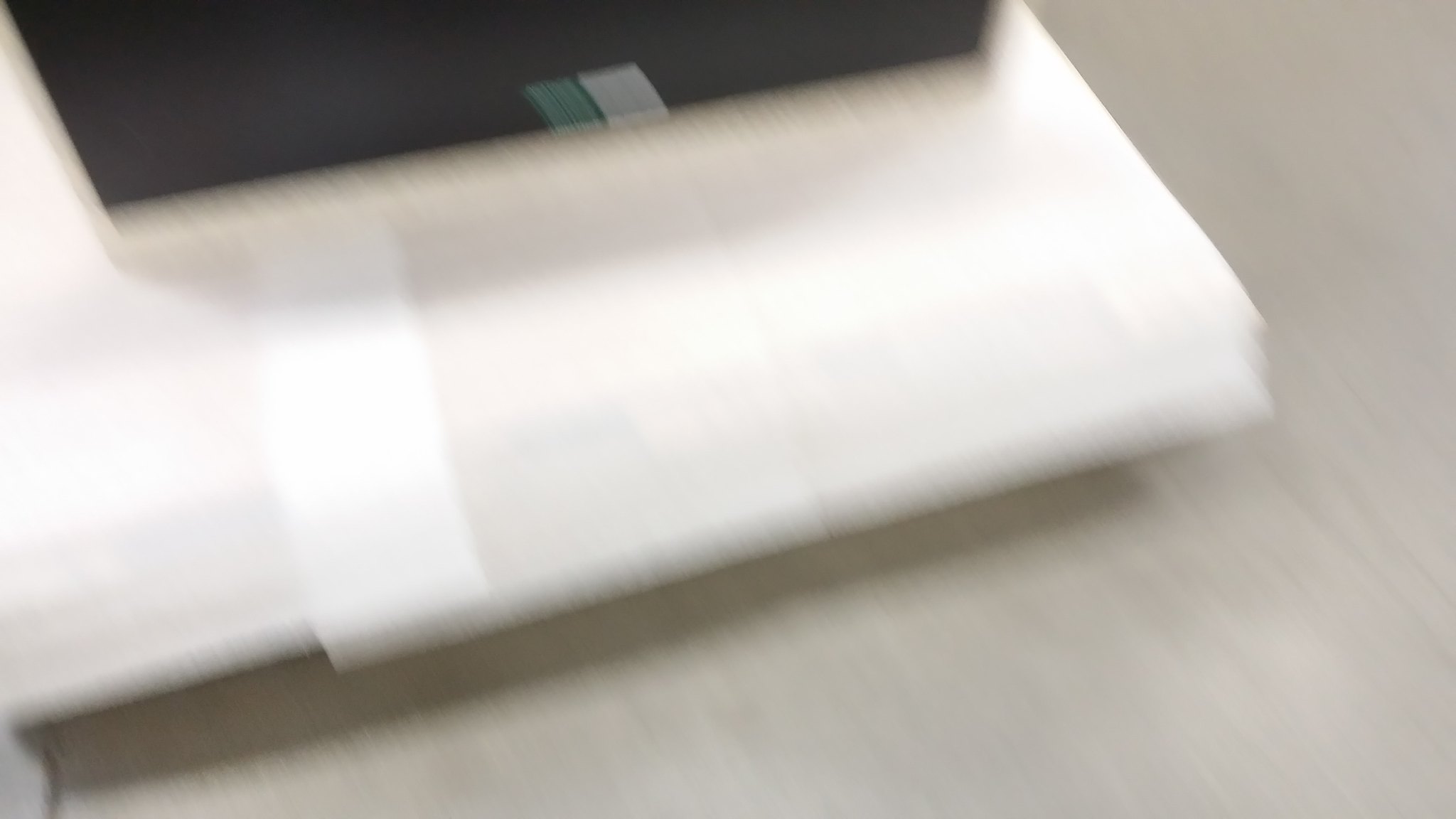A close-up, slightly blurry image shows a flat, white object that appears to be a folded curtain or a bolt of sheer white fabric, resting on a beige counter or table. In the middle of the fabric, there is a thicker white hem. On top of this fabric, a black box is placed, with a small tab of a green and gray ribbon emerging from beneath it. The lighting casts shadows of both the black box and the white fabric onto the surface below, adding depth to the scene.